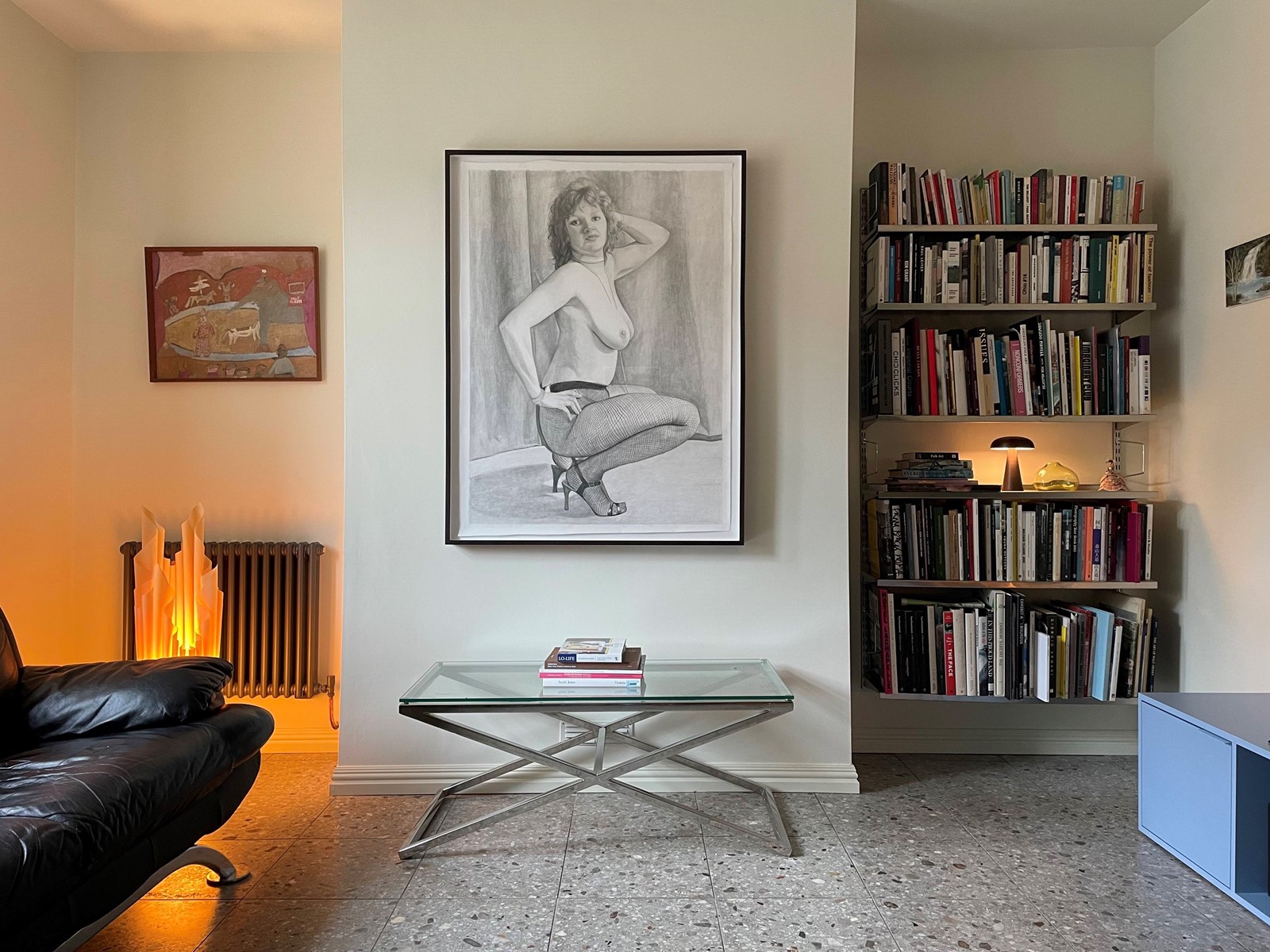The image captures a cozy and eclectic living room divided by a central wall or wide pillar. On the left side, there is an old-fashioned radiator with a framed picture above it, and a black leather couch in front of a lamp. To the right, the wall showcases two sets of overfilled book shelving with various books, tchotchkes, and a small stack of books on a small table. Adjacent to the bookshelves is another picture and a distinctive blue table.

The focal point of this room is the central divider, which displays a large pencil or charcoal drawing of a nude woman crouched down, posing provocatively with stiletto heels and pantyhose. Her left arm is raised, with her hand placed in the middle of her head, while her right hand rests on her hip. Below this striking artwork is a chrome and glass table topped with a stack of books, adding to the room's artistic and intellectual atmosphere.